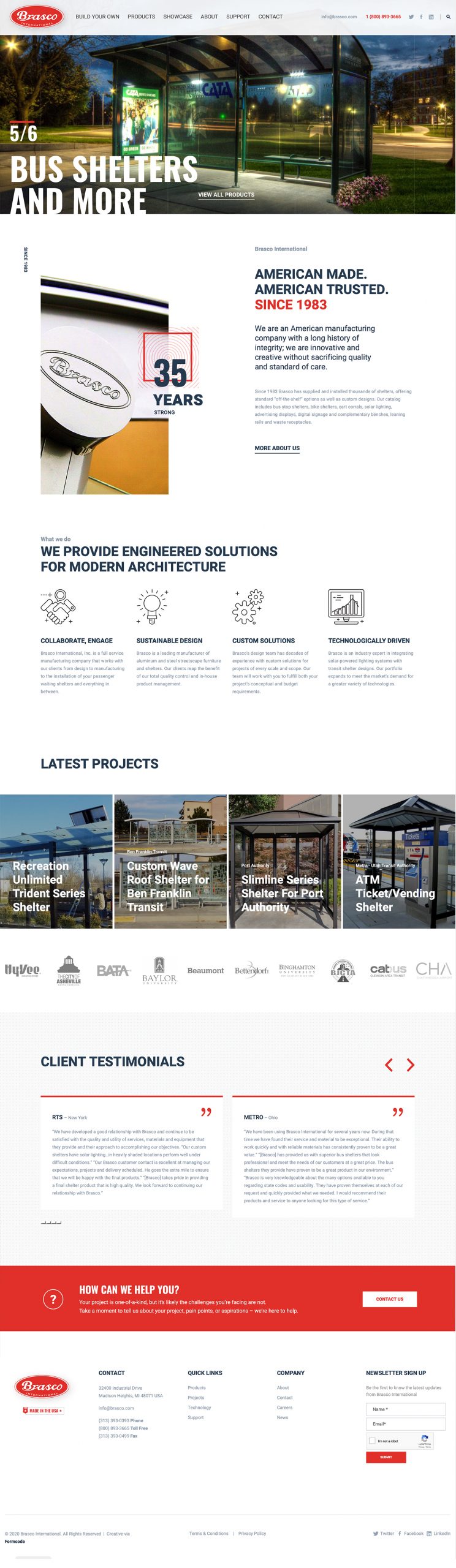This screenshot captures the homepage of a website with a predominantly white background. At the very top, a pale gray bar spans across the page. In the top left corner, there is an oval red logo, followed by a navigation bar offering six options and a potential search feature.

The header image showcases a bus stop at night, featuring the text "Bus Shelters and More" in white. Below this, a predominantly white section displays. Prominently, there is a photograph of a logo, which includes the text "35 Years" beside it. The headline next to the photograph proclaims, "American Made, American Trusted Since 1983," with a smaller print underneath.

Further down, a bold black heading introduces a section, but the text is too small to decipher. Below this heading, four columns are presented, each topped with a line drawing. The section titled "Latest Products" appears next, highlighted with a dark navy background and accompanied by four clickable thumbnails.

Beneath this, a selection of logos presumably representing suppliers or featured products are displayed. Near the bottom, a pale gray block contains two white boxes with client testimonials, underlined in red. Following the testimonials, a red block extends across the width of the screen, featuring white text, and the oval red logo reappears on the left side.

Finally, the bottom of the page is organized into four columns likely containing sections such as "Contact Us," "About Us," and "Information." The very bottom of the screen includes some text relating to the website.